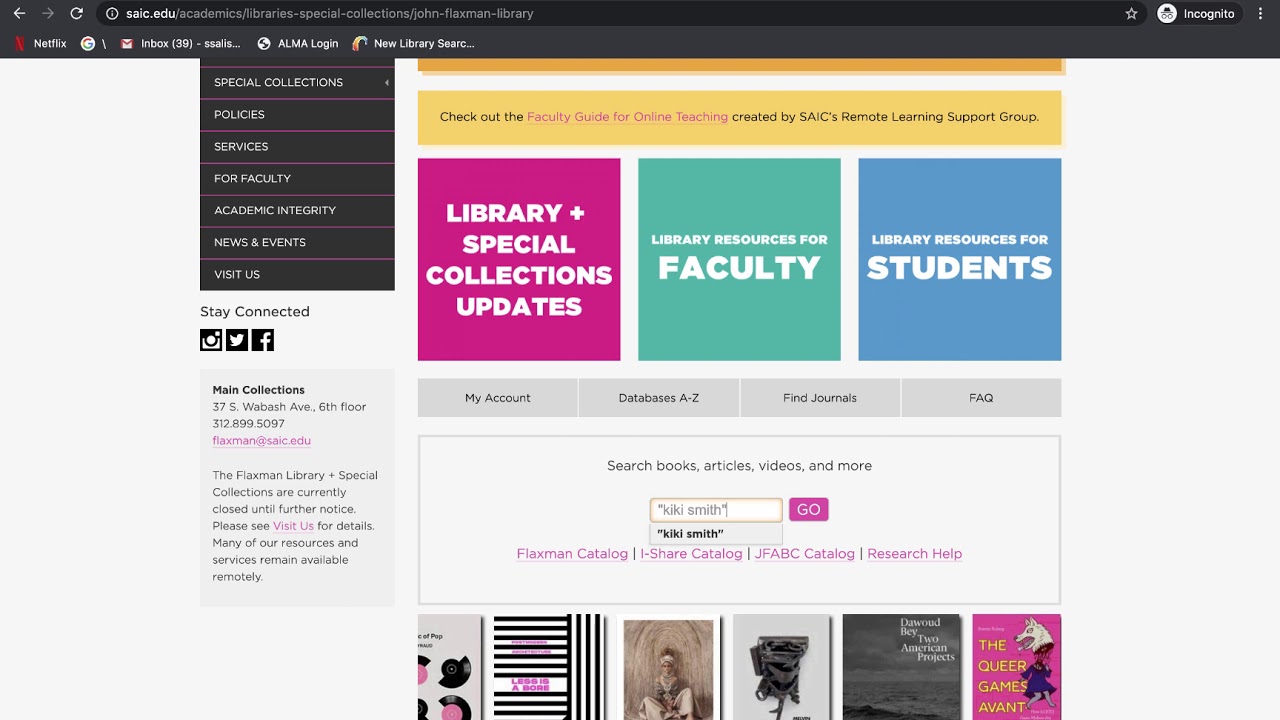The image features a complex and colorful layout. 

At the top, there is a large gray rectangle containing a smaller black rectangle, both filled with white text and symbols. Just below, a red icon is juxtaposed with additional white text and symbols, which are difficult to distinguish. Following this section, there is a dropdown box lined with purple, containing text between these lines. Beneath the dropdown box, black text alongside black symbols continues, ultimately leading to a line of purple text. 

A black paragraph follows, interspersed with purple lines. On the right side of the image, a dark orange rectangle is situated above a dark yellow rectangle, both containing a combination of black and red text. Further down, a pink square announces "Library + Special Collections Update," accompanied by a greenish square with "Library Resources for Faculty," and a blue square reading "Library Resources for Students."

Below these squares, a gray rectangle filled with text is displayed, followed by another gray-outlined rectangle with text, a yellow outlined rectangle with text, and a pink rectangle labeled "Go." Small pink text follows beneath this area. The image concludes with a series of pictures arranged at the bottom.